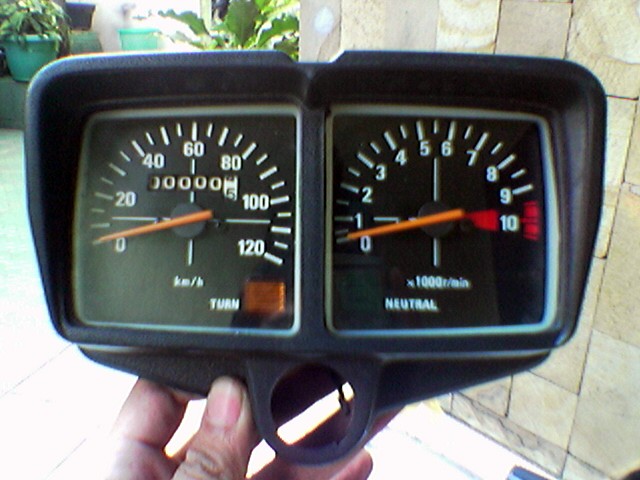The photograph captures a hand holding up an old-fashioned speedometer and odometer combination device, likely originating from the 1980s or 1990s. The speedometer, analog in design, has a display measured in kilometers per hour, ranging from zero to 120. The odometer readings on the device are at zero, indicating either a lack of use or a recent reset. Adjacent to the speedometer, the right side features a tachometer that measures up to ten times revolutions per minute (R x 10 RPM), with indications for gear positions including neutral. The backdrop consists of a stone marble wall, suggesting the image was taken outdoors, possibly in a courtyard. The setting is further embellished with greenery, including potted plants, adding to the casual, almost nostalgic atmosphere. The photograph itself has a slightly grainy texture, typical of images from several decades ago, striking a balance between nostalgic clarity and the passage of time.